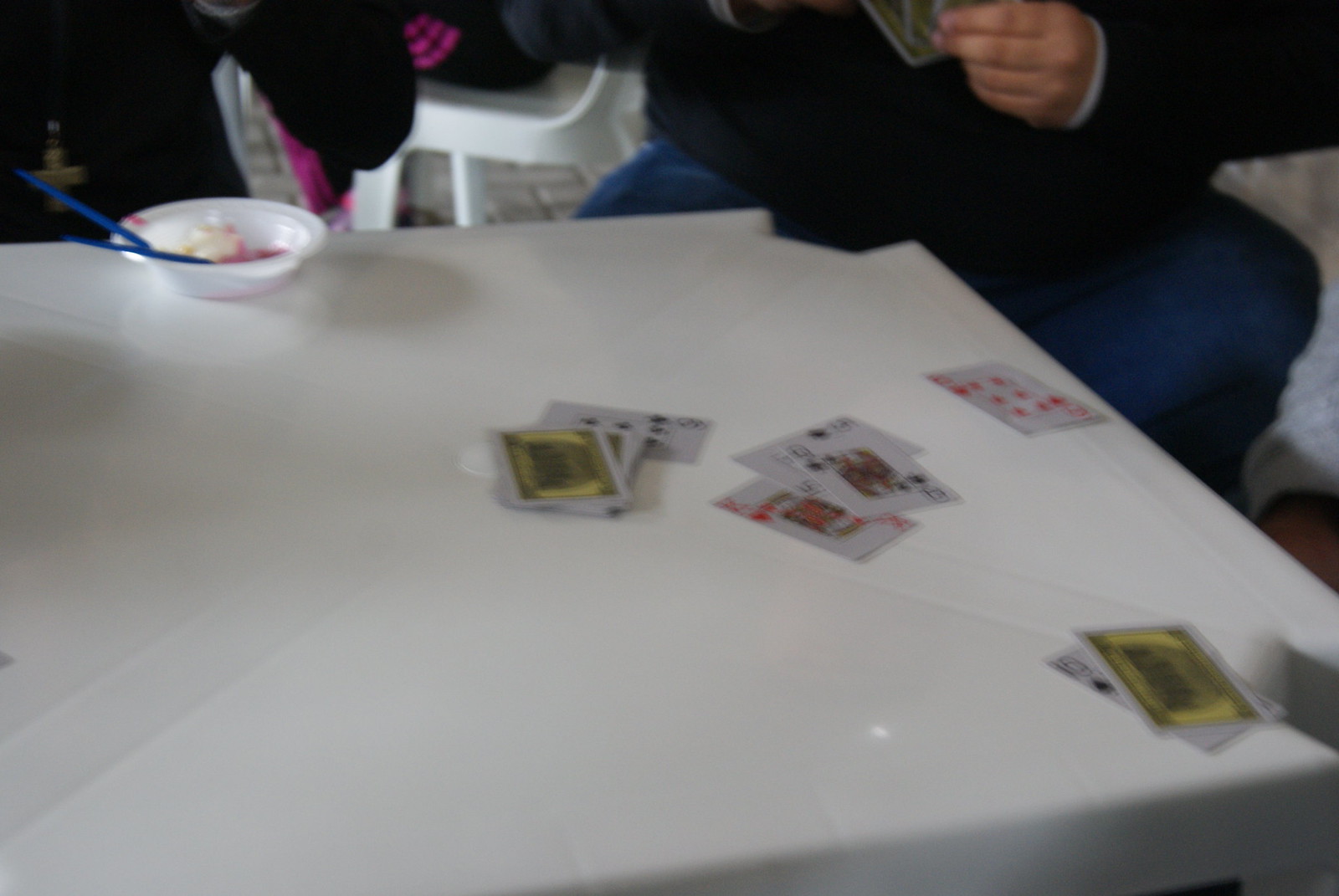In this overhead image, we see a lively card game in progress on a pristine white table. Three distinct piles of cards and a single card are spread across the table, indicating an ongoing game. Near the upper part of the table, there's a bowl containing a dessert, possibly cake, adorned with two blue utensils that could either be straws or forks. Dominating the scene, a large gentleman is seated at the table, clad in a black sweater and blue jeans. His hand is visible, holding several cards, clearly participating in the game. He is seated on a white plastic chair matching the table. In the upper left background, a young girl is kneeling down, sporting black sweatpants with a pink Adidas logo. The deck of cards being used in the game appears to be standard, with the card backs featuring a distinctive yellow design. This indoor scene captures the essence of a casual and engaging card game among friends.